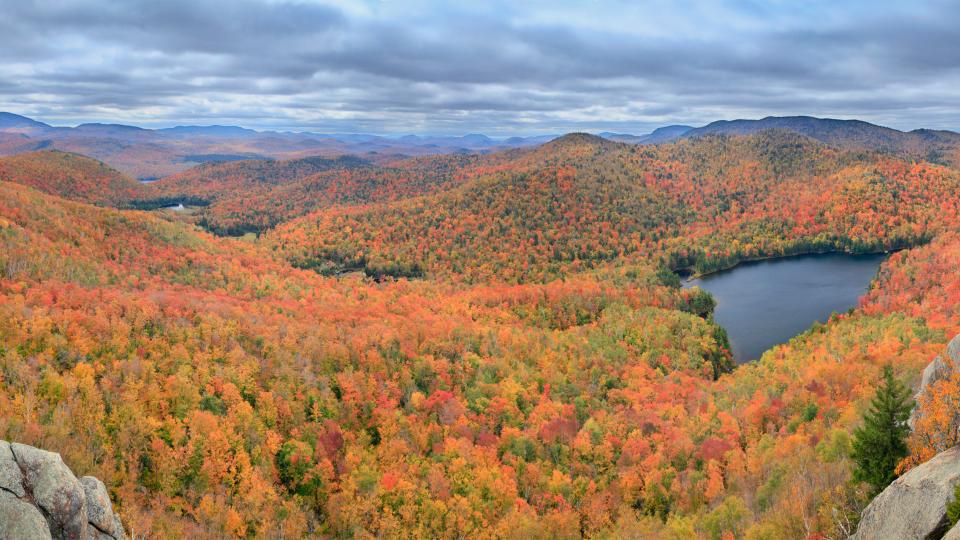This is a detailed landscape photograph of hilly forest land in the fall, capturing the vibrant interplay of nature's colors. The scene is dominated by an expanse of trees, displaying a palette of oranges, yellows, reds, and greens that stretch from the foreground to the distant horizon. These hues create a striking contrast with the cloudy sky above, which dominates the top 20% of the image with dark gray clouds hinting at imminent rain, yet the foreground appears sunny.

Rolling hills or mountains form a picturesque backdrop, their peaks appearing blue from a distance, suggesting stone-topped summits. Interspersed among the trees are bodies of water with dark blue hues, possibly a pond, lake, or river, whose course meanders through the landscape but is partially obscured by the hills.

In the bottom left and right corners, gray cracked boulders add a rugged texture, with a solitary pine tree visible on the right-hand side. The middle of the image on the right also features a noticeable waterway, contributing to the serene and nature-oriented ambiance. The photograph showcases a mix of clear valleys and forested hills, presenting an exquisite and immersive view of this autumnal, nature-rich area.